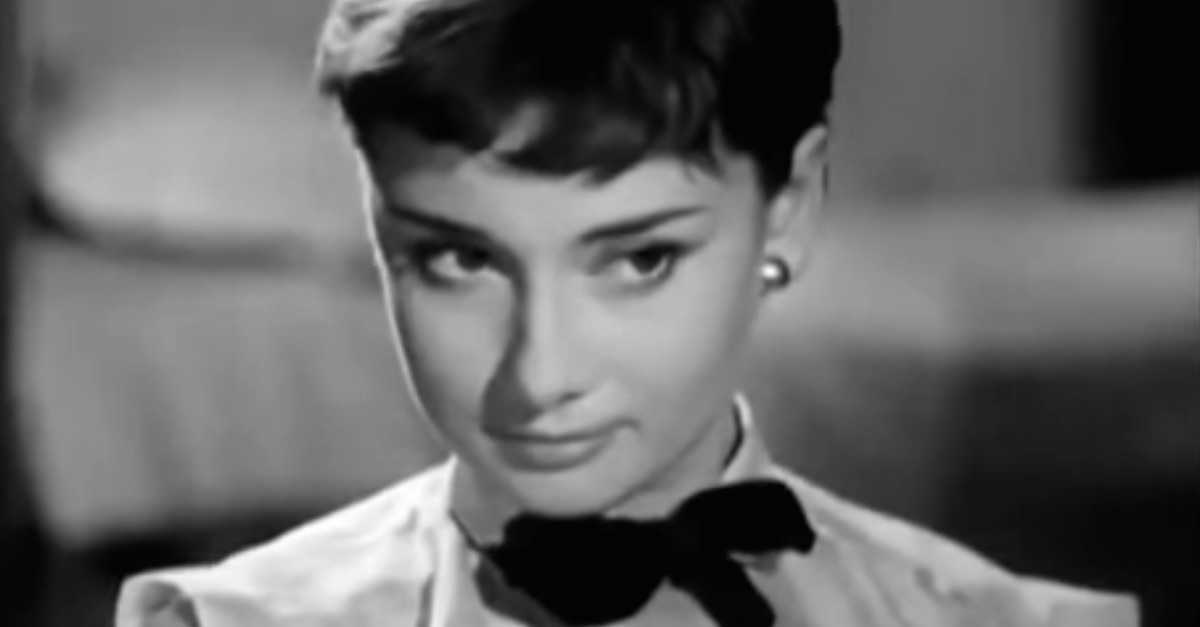In the black and white image, a woman resembling Audrey Hepburn is gracefully captured in a close-up. She is adorned in a crisp white shirt paired with a black bow tie. Her hair is styled in an elegant updo, showcasing a prominent earring on her left ear. She gazes slightly to the side with a composed expression, her thin nose and pursed lips forming a subtle half-hearted smile. The background is gray and black, appearing hazy and blurred, further emphasizing her timeless and classic beauty. The overall composition, with her dark eyes and eyebrows adding depth, evokes a sense of vintage elegance.